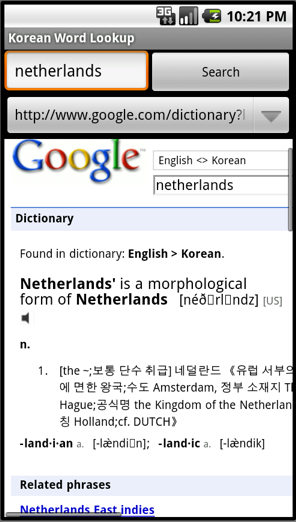This image displays a screenshot taken on an Android phone, as evidenced by the recognizable Android icons. The screenshot captures a Google search conducted on a Korean language lookup website. In the search box, the user has entered "Netherlands" in an attempt to translate it from English to Korean. The Google logo is prominently visible in the top left corner, confirming the use of Google for the translation. Alongside the main translation query, a related phrase "Netherlands East Indies" is also shown. The phone's status bar reveals that it is connected to a 3G network with 2 out of 4 signal bars and is currently charging at approximately 50% battery life. The time displayed on the phone is 10:21 PM.